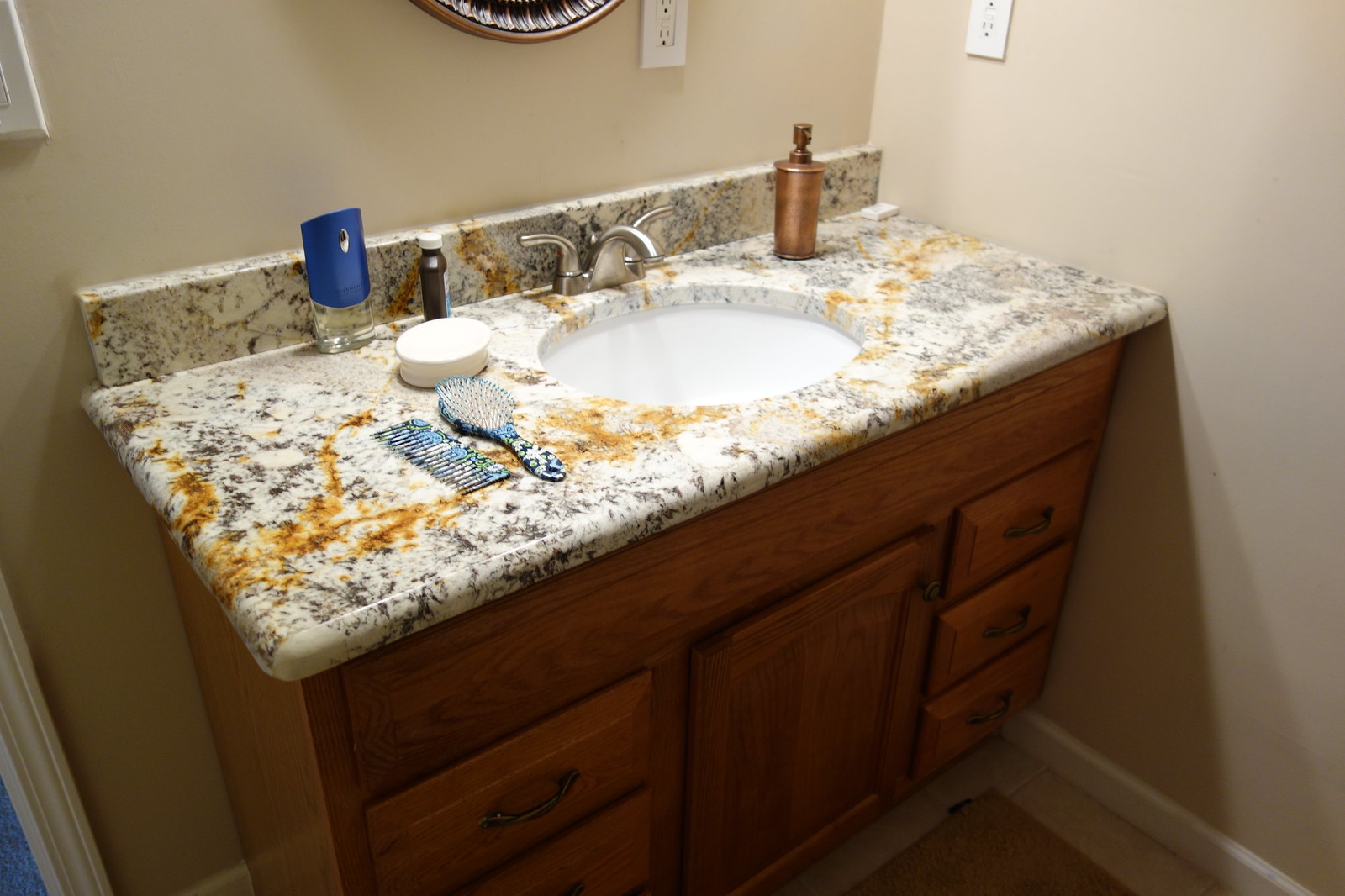A meticulously detailed photograph captures a sophisticated bathroom vanity setup. The focal point is a wooden vanity with an elegant medium-toned, orange wood finish. Its extended design features a central sink flanked by spacious dual side counters, topped with a luxurious granite countertop. The countertop boasts an intricate pattern of black, white, gray, and rust-brown hues, complementing the sleek, silver faucet at the sink's center.

On the vanity, from right to left, a collection of carefully arranged items can be seen. A small bar of hand soap sits in the far-right corner, alongside a weathered brass soap dispenser. A comb and brush set, crafted in heavy-duty plastic with a striking light blue, white, and black speckled design, are positioned next. An oval bar of soap and a petite brown bottle with a white cap, resembling a medicine bottle, add to the assortment of personal care items. Lastly, an air freshener or hand sanitizer dispenser with a clear base and blue top, featuring a spray opening, completes the array.

The backdrop consists of two cream-colored walls, subtly framing the vanity. The L-shaped layout of the walls places the vanity towards the right side of the room while remaining central within the frame of the image. Above the vanity, two white outlets with dual plug sockets are visible, and the very bottom edge of a round mirror is just discernible. The vanity's design includes a large, false drawer along the top, a central cabinet, and three drawers on either side of the cabinet, showcasing both form and function in this elegantly detailed bathroom setting.